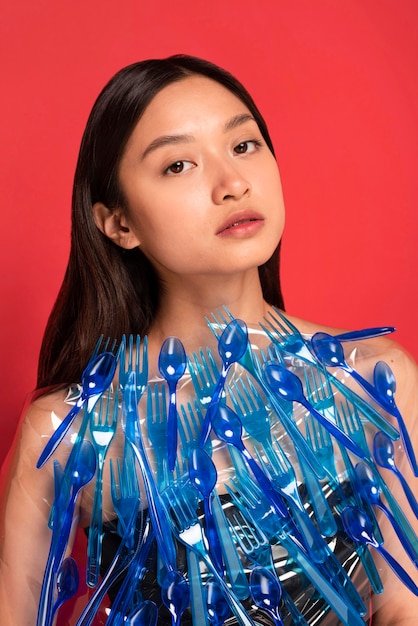In this striking image, we see a young woman standing against a vivid red background. She has long dark hair, parted in the middle and pulled back behind her ears, complementing her clear, brown eyes and subtly made-up face. Her expression is serious, with slightly agape lips accentuated by red lipstick that harmonizes with the backdrop. The focal point of her attire is an avant-garde dress made of various pieces of blue plastic cutlery—spoons, forks, and knives—arranged intricately along her shoulders and chest. The cutlery appears to be held together by a clear cellophane-like material, adding a unique artistic element to her outfit. Although we only see the upper part of her body, the detailed composition and unconventional materials make the image a thought-provoking piece of art.